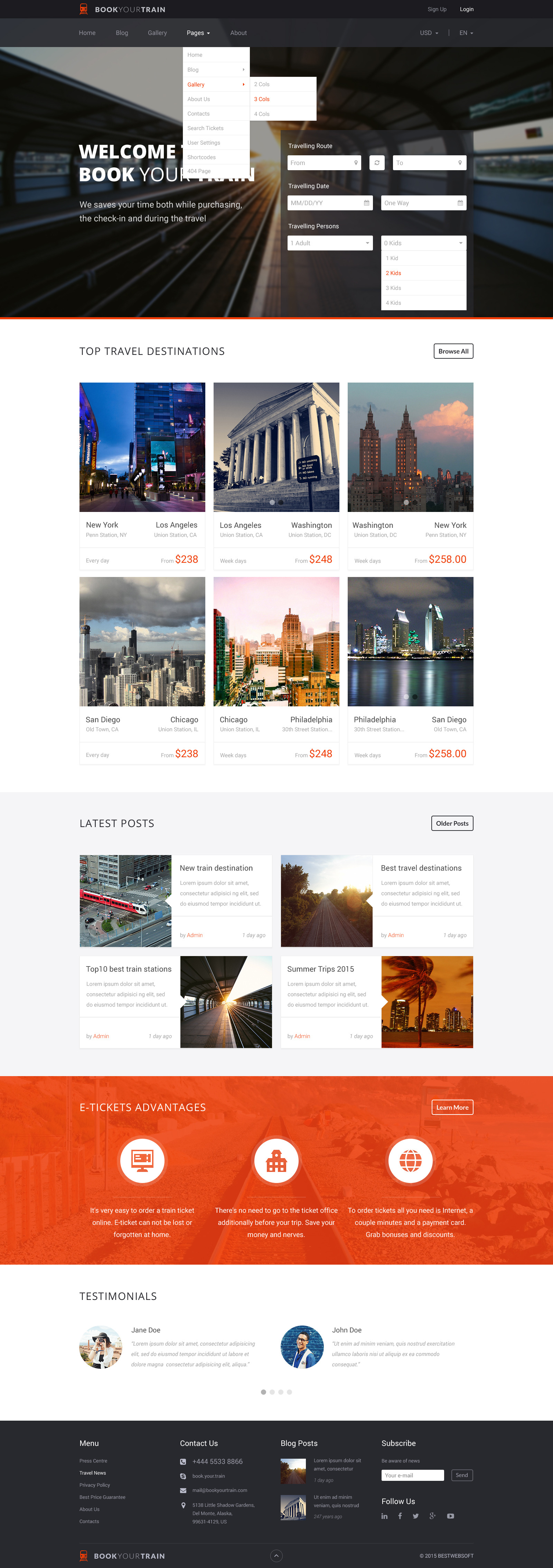This image depicts a hotel booking webpage. At the top, there is a navigation bar with seven options, although the small text makes it difficult to read the brand name. An individual is currently active on the fourth link from the left on this top bar. In the center of the page, a welcome message is partially obscured by the navigation bar. Beneath this, the text reads "Book your review," accompanied by fields likely intended for entering dates or locations for booking.

Further down, the webpage showcases "Top Travel Destinations," with cities such as New York, Los Angeles, Washington, San Diego, Chicago, and Philadelphia listed. The text is somewhat challenging to decipher. Below this section are headers for "Latest Post," "E-tickets and Advantages," and "Testimonials."